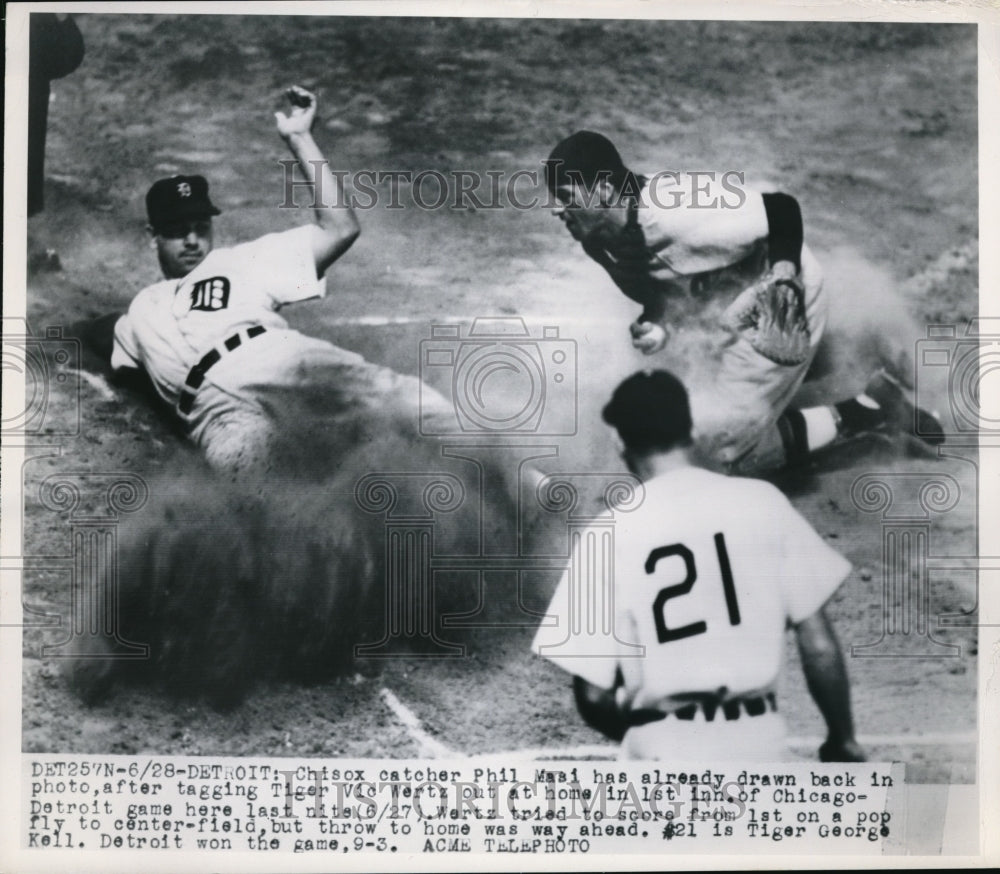This is a square, black-and-white photograph that appears to be clipped from a newspaper, likely from the late 1940s or 1950s, capturing a dramatic moment in a Major League Baseball game between the Chicago White Sox and the Detroit Tigers. The scene shows a Detroit Tigers player, Vic Kurtz, sliding into home plate in an explosion of dust while Chicago catcher Phil Maia stands aside with the ball in his hand, having apparently completed the tag. Another player is seen standing and looking down at the contentious play, which has obscured the base in a cloud of dust. The photo includes a caption reading: "Chicago catcher Phil Maia has already drawn back in the photo after tagging Tiger Vic Kurtz at home," and features a watermark that says "historic images" alongside icons of cameras and Greek columns. The darkened field and visible baselines highlight the central action, making this a memorable and controversial moment preserved in the sports section of a newspaper.